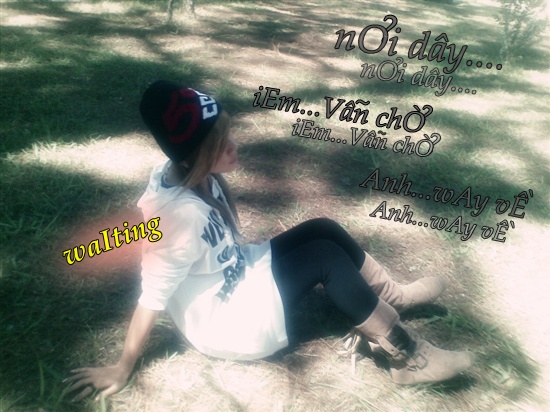In a serene outdoor setting, a young person sits on the dirt, partially shaded by the dappled light through the trees. She is wearing brown, mid-calf boots with straps on the sides, black tights, and an oversized white hoodie adorned with blue lettering. A black beanie with white and red graphics covers her head, and long brown hair partially obscures her face, cascading down to her chest. Her right arm, which is visible, has the sleeve pulled up to her elbow, revealing white fingernail polish and a ring on her index finger. The image is accented with several textual elements: yellow text on the left side that reads "Waitink," and repeated lines of letters in the top right corner that spell out N-O-I-D-A-Y, E-M-V-A-N-C-H-O, and A-N-H-W-A-Y-V-E. The background has a blurry, glossy filter, enhancing the tranquil yet mysterious ambiance of the photograph.